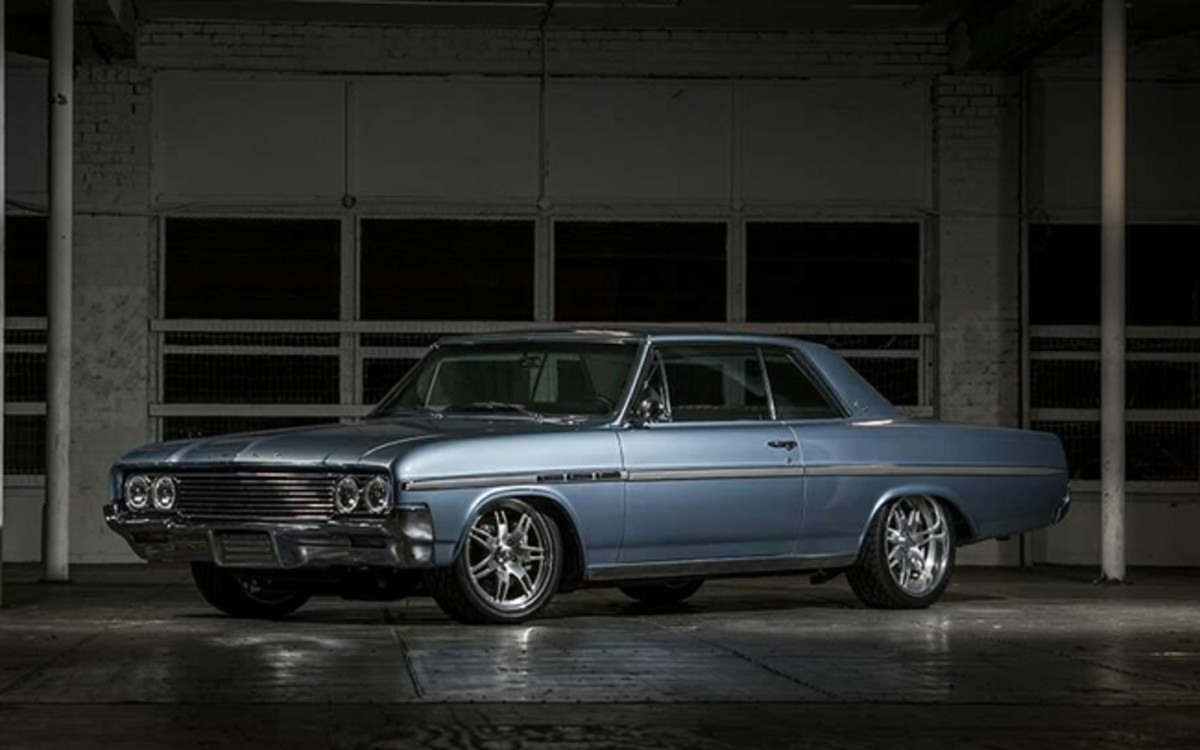This detailed caption combines the key shared and unique elements from the three inputs:

---

This photograph features a beautifully maintained vintage car, possibly of European make, parked in an immaculately kept display garage. The car is a striking light blue, almost a dusty or steel blue shade, with a high polish that captures the light. Its sleek design includes a chrome grille adorned with dual headlights on each side and a raised silver metal stripe running along the length of the body, adding a stylish touch. The car sits low and is missing a license plate, though a designated area for one is visible. It also boasts custom hubcaps and extensive chrome detailing around the wheels and grille, accentuating its luxurious appearance.

The setting—a spotless, well-organized garage—further highlights the car's prominence. The garage has a bank of windows and what appears to be raisable doors, likely part of a concrete or brick structure, illustrating a mix of functionality and aesthetic appeal. Spotlights aimed at the car enhance its features and suggest it is a prized possession, possibly belonging to a collector or an affluent individual. The absence of tools and the clean environment emphasize its display status rather than day-to-day use.